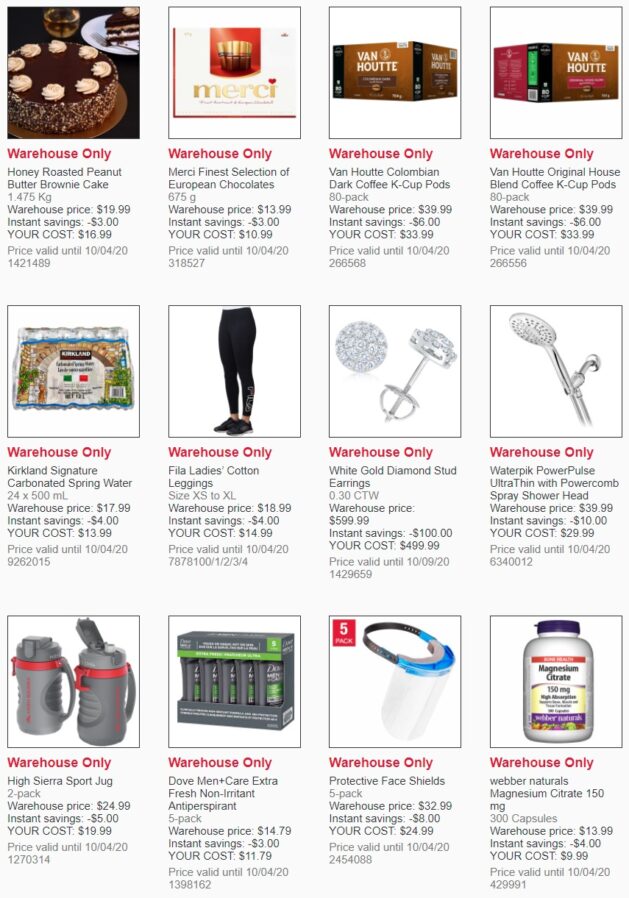The image is a vertically oriented advertisement layout, taller than it is wide, featuring 12 distinct items in a grid-like arrangement. Each item occupies a rectangular section divided into two squares: the top square for an image and the bottom square for descriptive text. 

1. **Chocolate Cake:**
   - Text: "Warehouse Only," "Honey Roasted Peanut Butter Brownie Cake."
   - Details: Weight, warehouse price, instant savings, customer cost, and price validity period are provided.

2. **Candy (Reese's Peanut Butter Cup-like):**
   - Image: Candy shaped similar to Reese's Peanut Butter Cups.
   - Text: Descriptive information about the candy.

3. **Colombian Coffee K-Cups:**
   - Image: Coffee pods labeled as Colombian coffee.
   - Text: Description and details on the product.

4. **General K-Cup Pods:**
   - Image: Assorted K-Cup coffee pods.
   - Text: Product details.

5. **Carbonated Spring Water:**
   - Image: Bottles of carbonated spring water.
   - Text: Product description and specifications.

6. **Ladies' Black Leggings:**
   - Image: Black leggings for women.
   - Text: Product details including material and sizes.

7. **White Gold Diamond Stud Earrings:**
   - Image: Pair of diamond stud earrings set in white gold.
   - Text: Specifications and pricing information.

8. **Water Pick (Shower Head):**
   - Image: A water pick designed for use as a shower head.
   - Text: Product features and benefits.

9. **Sport Jug:**
   - Image: A large sports water jug.
   - Text: Description and capacity details.

10. **Soap:**
    - Image: Bar or container of soap.
    - Text: Product specifications and ingredients.

11. **Face Shield:**
    - Image: Protective face shield.
    - Text: Description and purpose.

12. **Vitamins:**
    - Image: Bottle of vitamins.
    - Text: Nutritional information and benefits.

Each item's section provides a concise yet detailed overview, including visual depiction and informative text detailing the product's key aspects, pricing, and availability.